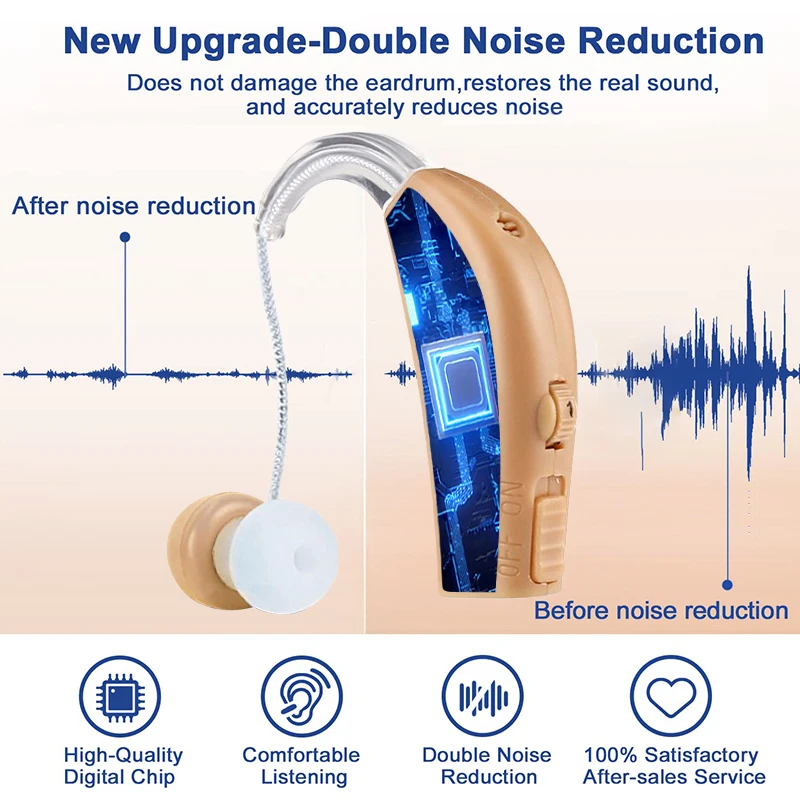This attention-grabbing advertisement for state-of-the-art noise-reduction earplugs or headphones showcases a sleek, modern design with a background transitioning from light pink to tan. Dominated by a close-up visual of the device, this ad intricately outlines the advanced technology within, symbolized by internal blue digital components. The central photograph reveals a flesh-colored hearing aid featuring intuitive controls, including a volume knob and an on-off switch, along with a clear earpiece designed for optimal comfort.

Above, bold blue text announces the "New Upgrade: Double Noise Reduction" feature, emphasizing that the device is gentle on the eardrums yet effective at restoring authentic sound and precisely diminishing unwanted noise. To the left, small sound wave lines with an arrow indicating "After Noise Reduction" contrast sharply with larger, chaotic lines on the right labeled "Before Noise Reduction," visually highlighting the aid's superior sound clarity.

Supplementary icons at the bottom, each circled in blue, reinforce key product benefits such as "High-Quality Digital Chip," "Comfortable Listening," "Double Noise Reduction," and "100% Satisfactory After-Sales Service," ensuring potential customers of the device's quality and user satisfaction.